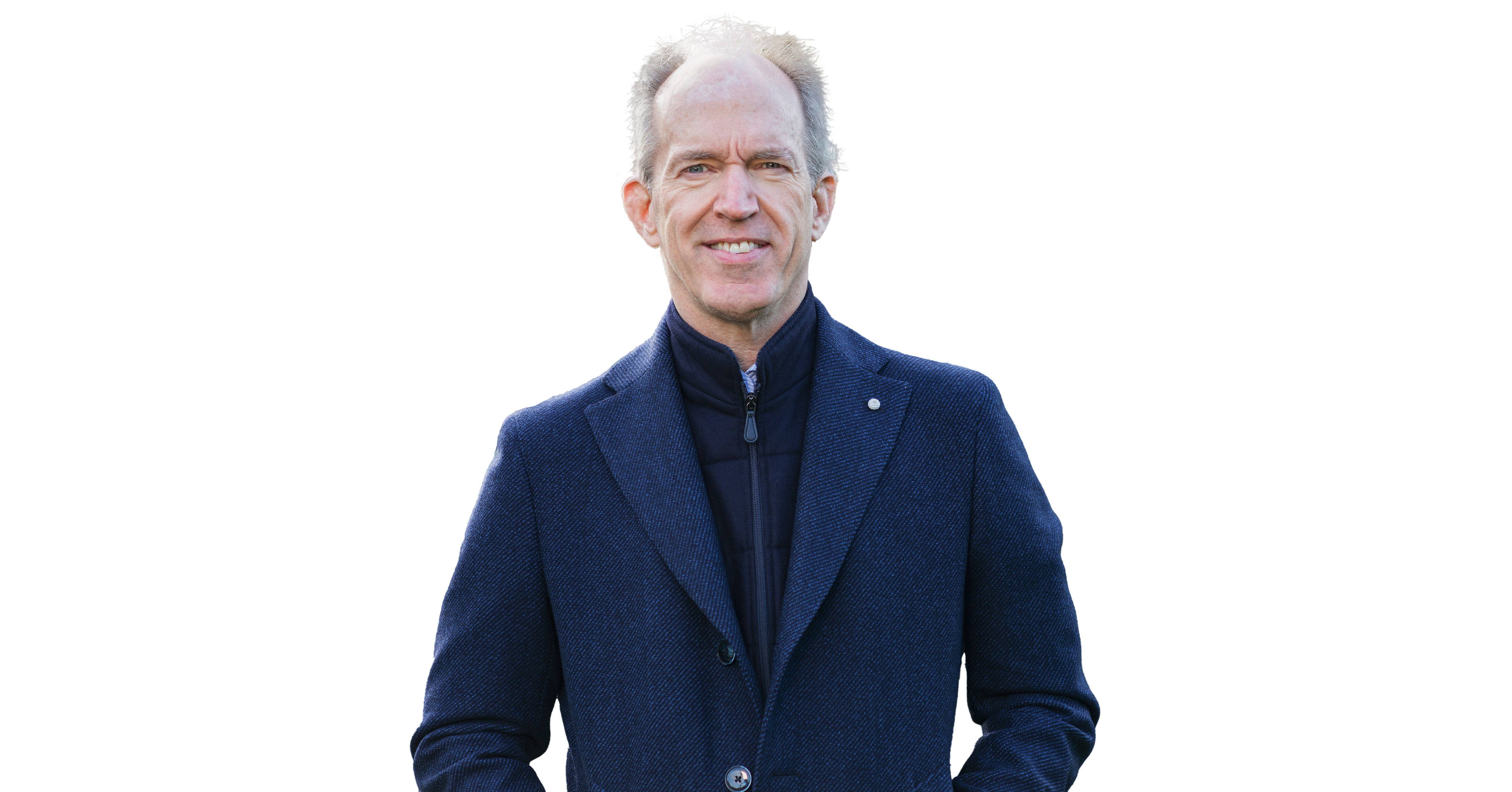This is a detailed portrait of an older Caucasian man with gray hair, where most of his hair remains on the sides while the top is balding. He has a familiar face that exudes a sense of wealth and celebrity, maybe suggesting he's an actor or musician. The man is smiling, revealing his upper row of white teeth. He is dressed in a sophisticated manner, wearing a navy blue tweed-style peacoat over a blue high-collared, zipper-up jacket that appears to have horizontal stripes, possibly resembling a puffer jacket. Additionally, there seems to be another layer underneath, potentially a button-up shirt. His overall appearance is elegant and stylish. The portrait has a plain white backdrop, emphasizing the man's features and attire without any distractions.